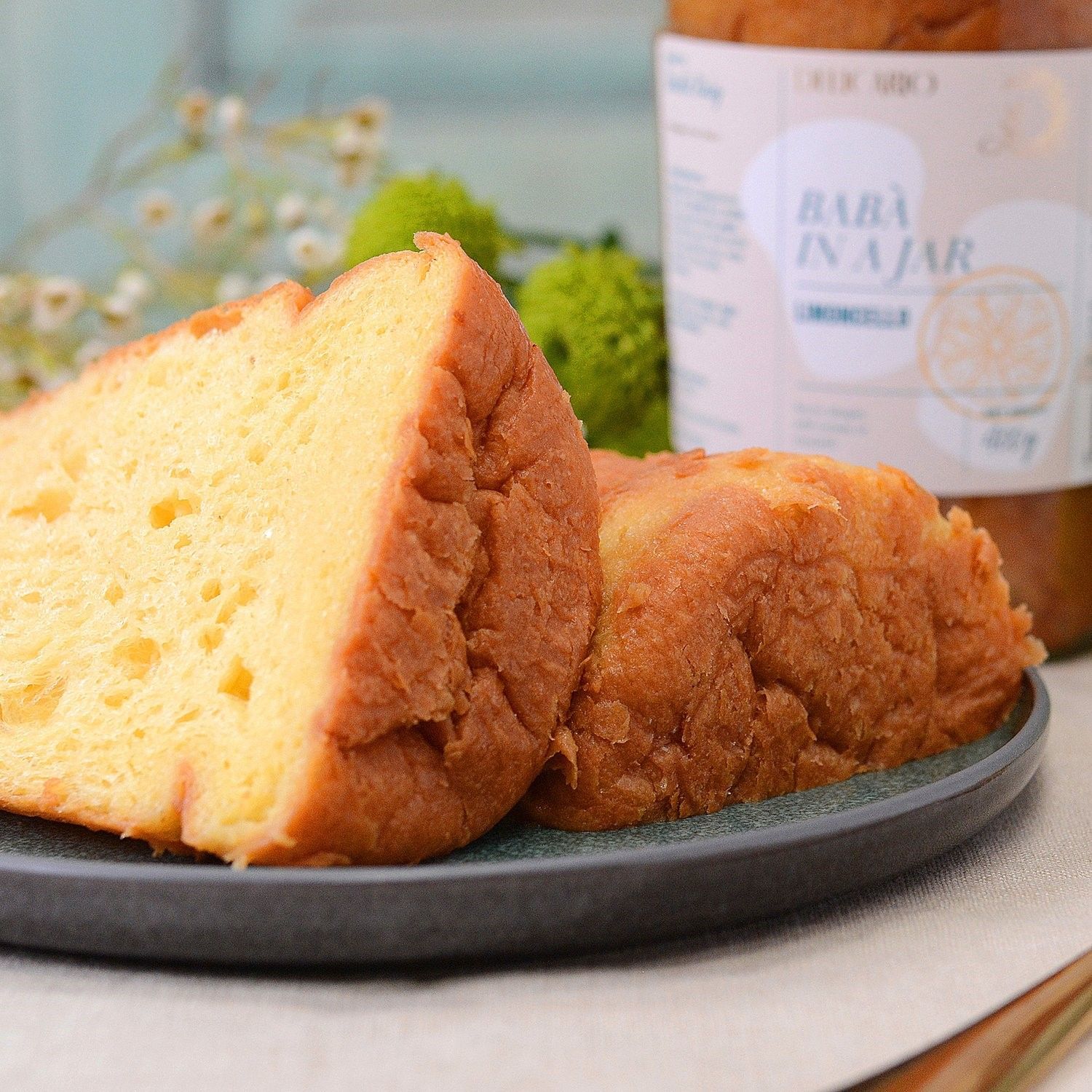The image shows a close-up of a brown, golden-crusted loaf that appears to be carrot or banana cake, sliced lengthwise to reveal a yellow, spongy interior. The loaf is positioned on a flat, gray stone-like plate that sits on a pale table mat atop a light wood-colored surface. To the right of the sliced loaf, the other half is placed upside down, hiding the yellow interior. In the background, there is a cylindrical jar with the label "Baba in a jar" in blue text against a white backdrop. The jar contains an orange substance that might be yams or jam. Surrounding the main focus, there are green plants and possibly some flowers adding to the background scenery.